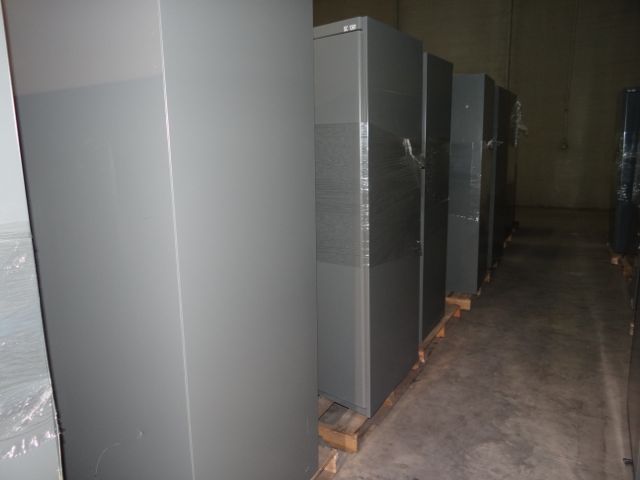The photograph showcases an indoor scene within a factory or storage room, featuring a row of tall, silver-gray refrigerators or metal cabinets neatly placed on wooden pallets. These storage units, wrapped around the middle with clear plastic, stand in an aisle-like formation reminiscent of supermarket rows. There are five visible cabinets on the left side, spaced approximately two feet apart, with another cabinet partially visible in the foreground. The floor below is a blend of light and dark gray and brown tones, resembling stained or marbled concrete. The far wall, discernible in the flash's illumination, appears to be a dark, muted green concrete surface. The overall picture captures the organized layout and reflective metallic quality of the units set against the subdued industrial room.